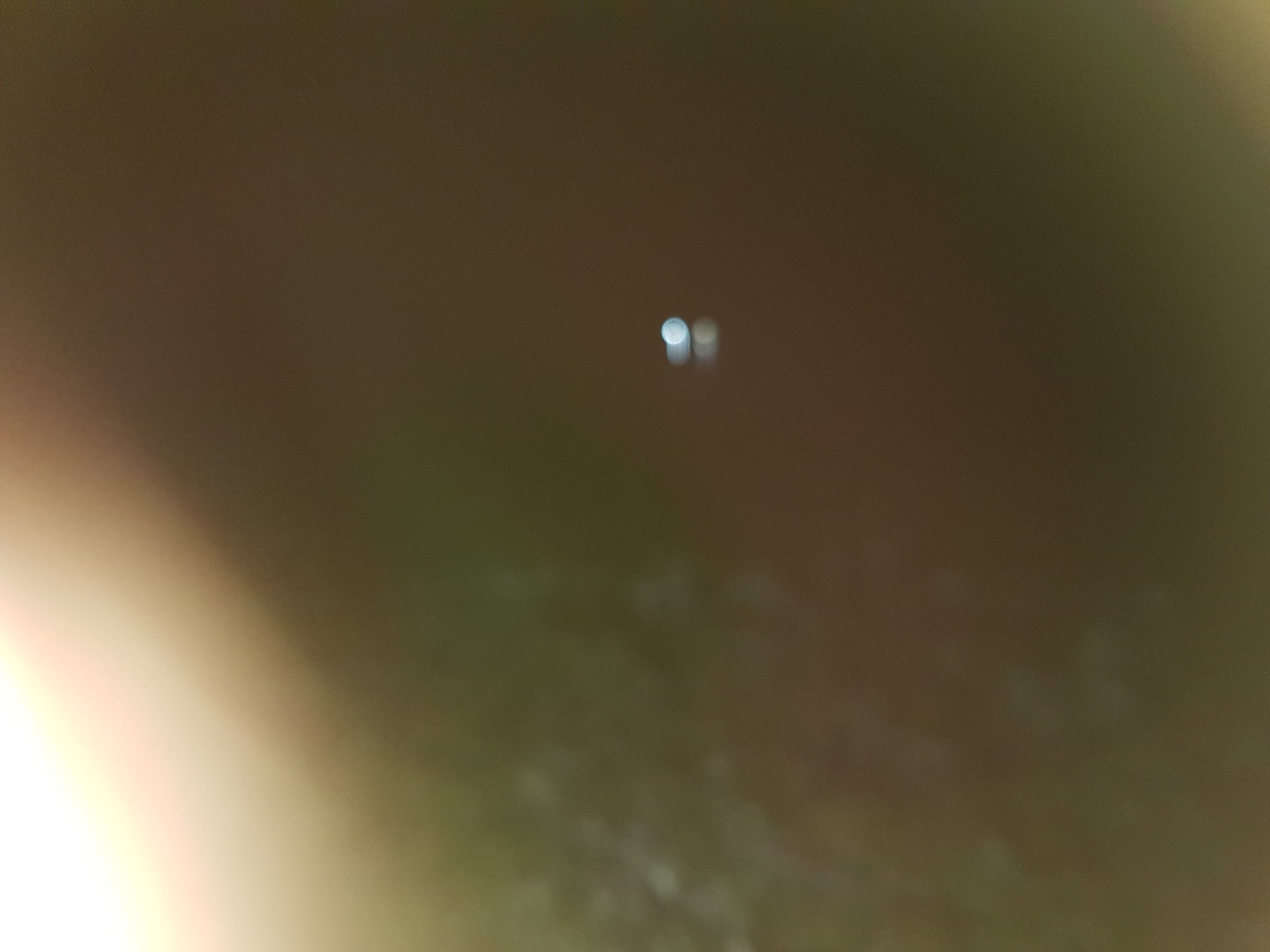A blurry nighttime photograph predominantly showcases a grassy area occupying the lower half of the image. In the center of the distant background, two round headlights are visible. The left headlight shines brightly white, while the right headlight, also white, appears significantly dimmer. Additionally, a very bright light is situated in the bottom left corner, gradually fading as it spreads out slightly upwards through the picture. The green hues of vegetation are faintly discernible amidst the overall darkness.